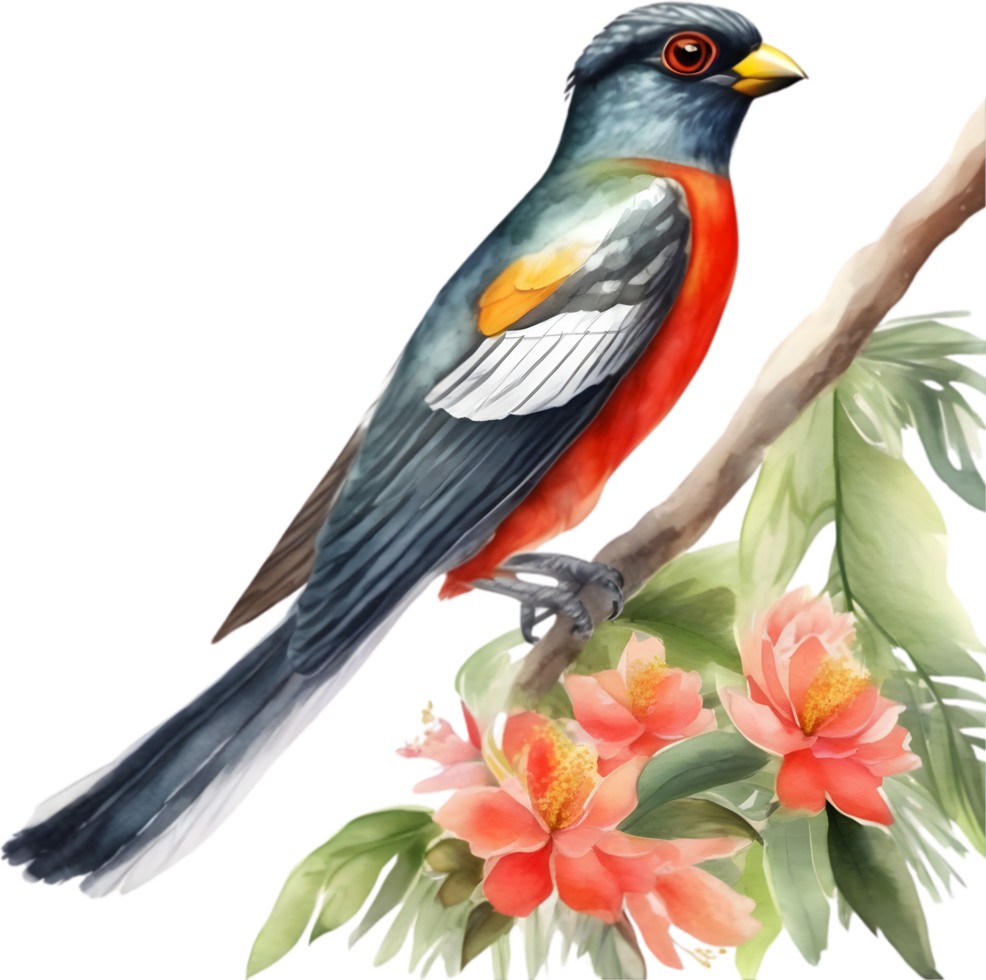In this detailed watercolor painting set against an all-white background, we observe a vibrant and unique bird perched diagonally on a brown branch. The branch, composed of both lighter and darker shades of brown, hosts an ensemble of green leaves and four pink flowers, each flower displaying delicate white highlights and vibrant yellow centers. The bird, facing the right side of the image with its beak closed, exhibits a captivating array of colors: its primary plumage is a combination of blue and gray, complemented by a red underbelly. The bird's wings showcase a mixture of white, yellow, and brown hues, with some black detailing. It has a yellow beak and striking red eyes, each containing a black spot. The bird's talons and claws are depicted in black, adding to its striking appearance. This intricate depiction, with emphasis on the multicolored bird and detailed flora, creates a vivid and enchanting scene.